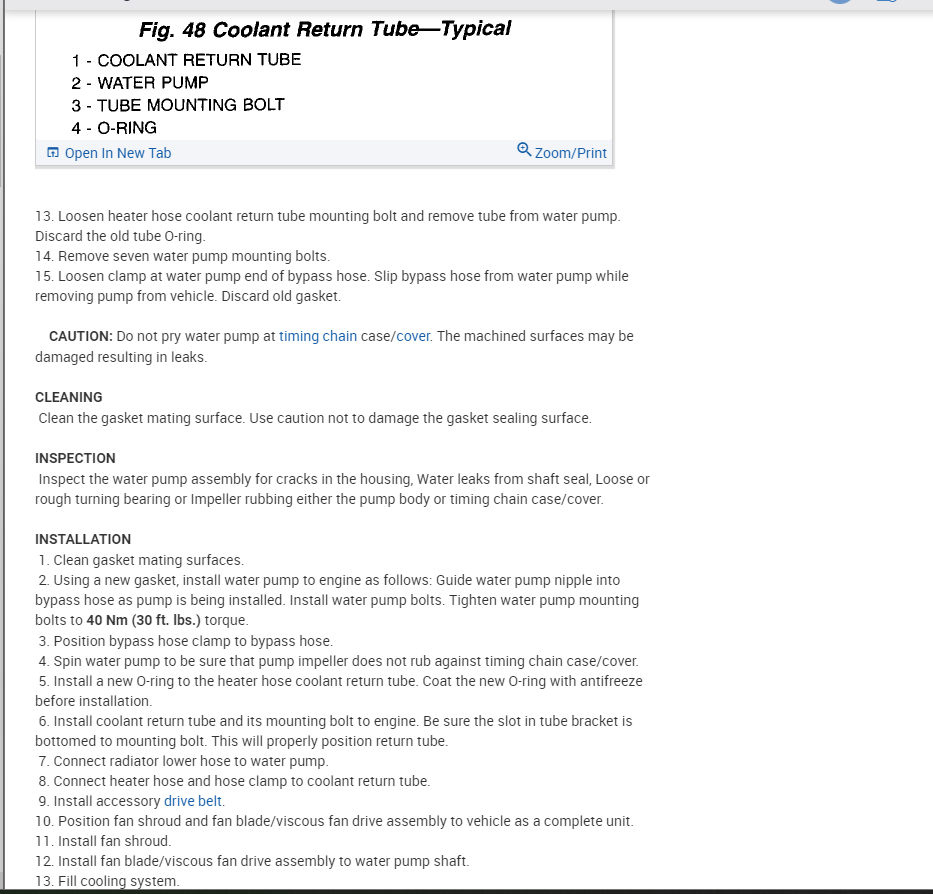**Detailed Caption:**

The image is a screenshot from an online instruction manual. The layout includes a thin line dividing the left and right sides, with a thin gray bar at the top. In the middle of the image, there's a labeled box titled "Figure 48: Coolant Return Tube (Typical)," which itemizes parts as follows:

1. Coolant return tube
2. Water pump
3. Tube mounting bolt
4. O-ring

To the side of the box, there are options to "Open a new tab" and "Zoom/Print."

The excerpt of the instructions provided starts with:

- Step 13: "Loosen the heater hose coolant return tube mounting bolt and remove the tube from the water pump. Discard the old tube O-ring."
- Step 14: "Remove seven water pump mounting bolts."
- Step 15: "Loosen the clamp at the water pump and bypass hose. Slip the bypass hose from the water pump while removing the pump from the vehicle. Discard the old gasket."

Additionally, there is a caution: "Do not pry the water pump at the timing chain case/cover; the machined surfaces may be damaged, resulting in leaks."

The subsequent sections include "Cleaning," which advises to "clean the gasket mating surface with caution to avoid damaging the gasket sealing surface," and "Inspection," which directs to "inspect the water pump assembly for cracks in the housing, water leaks from the shaft seal, loose or rough-turning bearing, or impeller rubbing against either the pump body or timing chain case/cover."

Highlighted in bold, the "Installation Instructions" consist of 13 steps. The first step reads "Clean gasket mating surfaces," and the final step instructs to "Simply fill the cooling system."